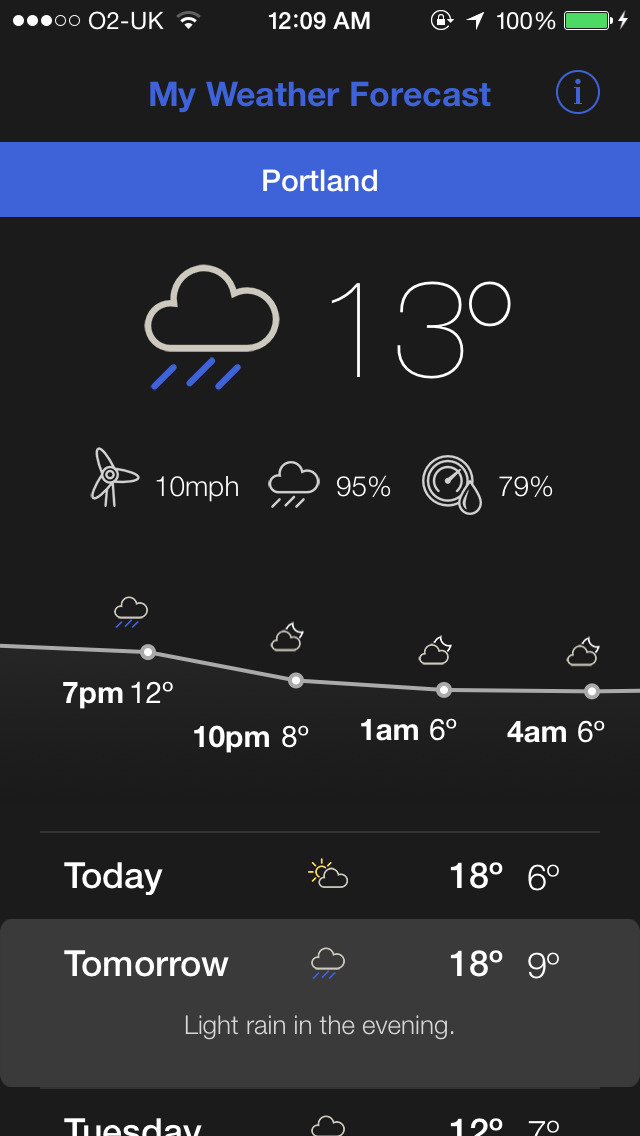This image is a screenshot of a cell phone currently displaying a weather application. The app is open against a black background. At the very top of the screen, there are five small horizontal circles, three of which are filled in white, and to their right, it indicates "02-UK." Centrally located, there is a Wi-Fi signal icon, flanked by "12:09 AM" in white text. On the rightmost side, white text features a padlock inside a circle, an upward arrow pointing to the one o'clock position, and "100% battery," with the battery symbol shaded green and a white lightning bolt to its right.

Below this, the screen transitions to a dark cornflower blue hue, displaying the title "My Weather Forecast" in bold white letters accompanied by a red circle with an eye icon. Within a solid blue banner stretching across the screen, it states "Portland."

The main body of the screen features a prominent white cloud icon with three diagonal blue rain lines, indicating rainy weather. Large white text below this shows "13°," while additional details below include a white fan icon labeled "10 MPH," signifying wind speed, and another cloud with white rain lines labeled "95%," indicating humidity. A gauge resembling an old car odometer with a raindrop icon and "79%" appears to signify precipitation probability.

Below this, a graph displays anticipated hourly temperatures along a diagonal line descending from left to right: 7 PM - 12°, 10 PM - 8°, 1 AM - 6°, and 4 AM - 6°. 

The forecast section features:
- "Today" in bold white letters, with an icon of a cloud partially obscuring the sun and temperatures listed as a high of 18° and low of 6°.
- "Tomorrow" with a simple cloud icon, temperatures of 18° high and 9° low, and a note of "light rain in the evening."
- "Tuesday" with another cloud icon in the center, and temperatures shown as 12° high and 7° low.